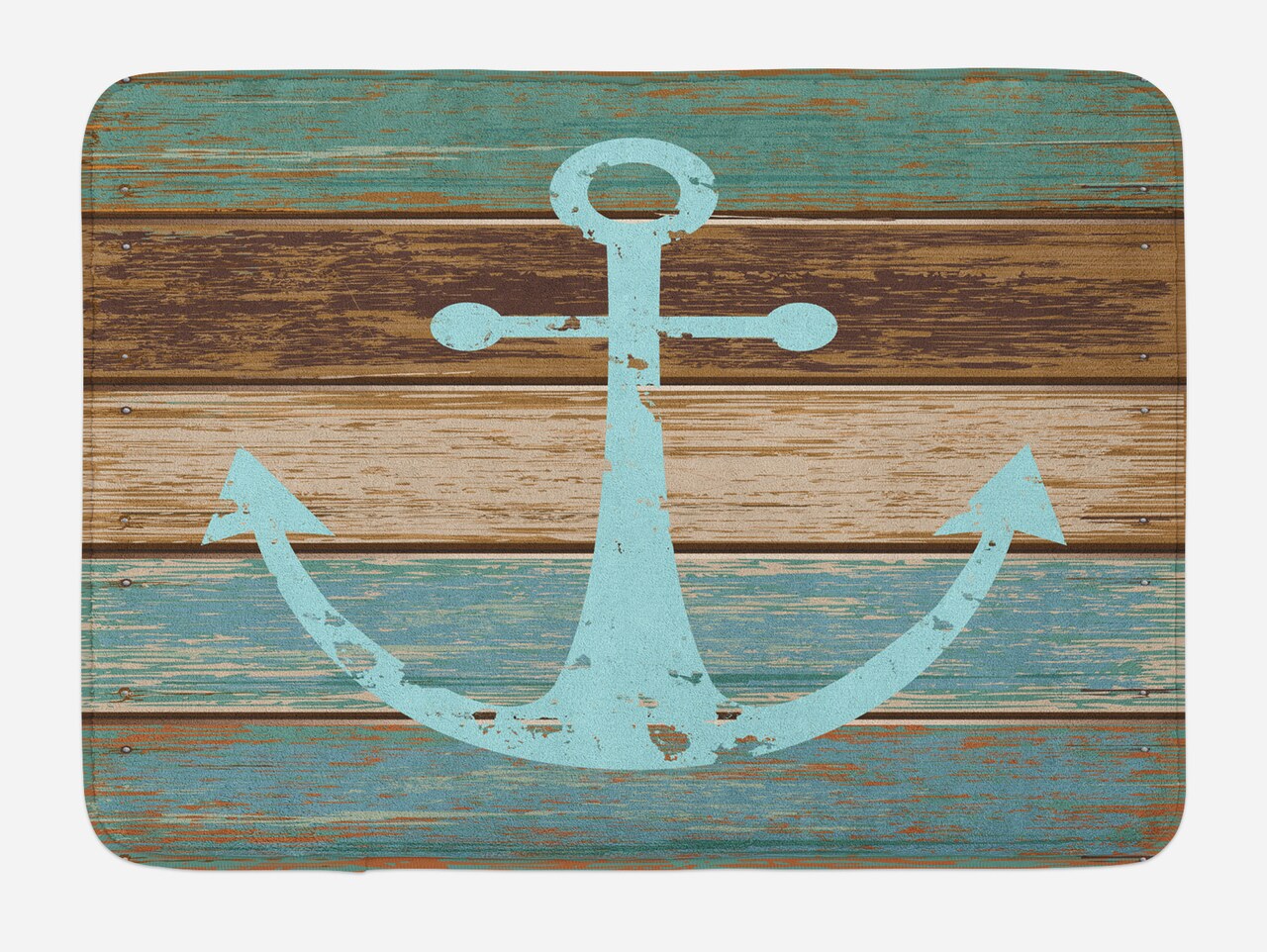This image showcases a vintage nautical-themed sign featuring a prominent blue anchor set against weathered wooden planks. The anchor itself, a Tiffany Blue with distressed elements that make it appear to have been scraped and worn, is centrally placed and stands out against the multi-hued wood background. The background wood displays a mix of aged and distressed shades, including periwinkle, cream, dark brown, and teal, enhancing the rustic aesthetic. The overall faded, worn look of both the sign and the anchor, with brown wood peeking through, reinforces the impression that the sign has been exposed to the elements over a long period. This richly detailed and textured image evokes a sense of maritime nostalgia, fitting perfectly in a nautical-themed bar or similar setting.